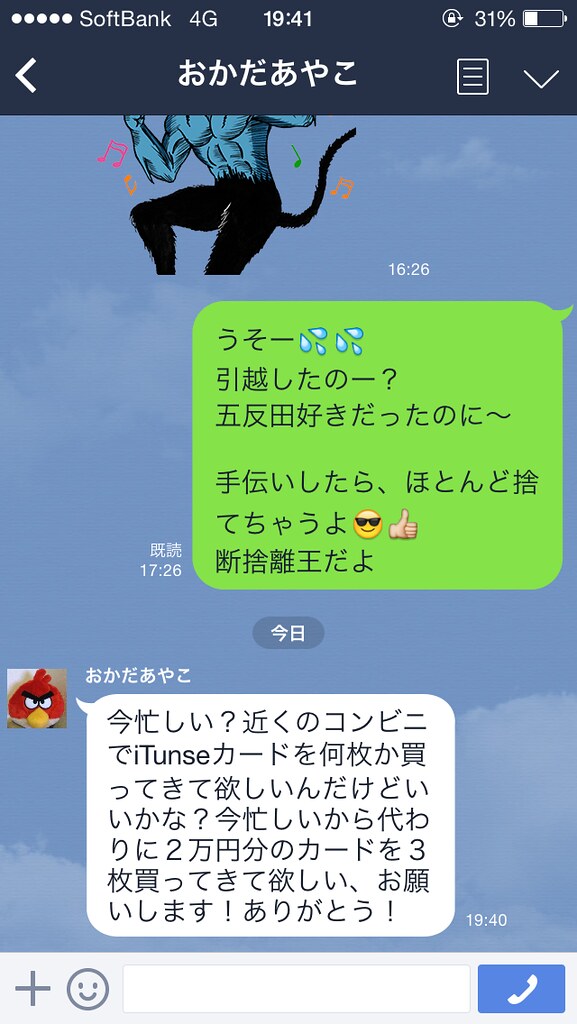The image is a screenshot of a cell phone messaging interface involving a dialogue in a language that appears to be either Japanese or Chinese. The top section of the screen is a navy blue header displaying the text "SoftBank 4G" at the top left, followed by five white dots. The time "1941" is centered, and the battery icon on the right shows 31% charge. Below this, there is an arrow pointing left, followed by some Asian characters, an icon of a page, and another arrow pointing down, all set against a blue background.

The messaging area starts with a partially visible cartoon figure, possibly a blue devil or a person with a cat tail, black pants, and no shirt, set against a blue and black background with musical notes. Below this, there is a green message bubble containing more Asian text and an emoji of a smiley face with sunglasses and a thumbs up.

Further down, the bottom third of the screen features an Angry Birds profile picture on the left, followed by another message bubble in a foreign language. The only recognizable text here is "iTunes." The very bottom row of the image includes a plus sign, a smiley face emoji, and a blue call button icon depicting a telephone receiver. Most of the screen background is a light blue, resembling a sky.